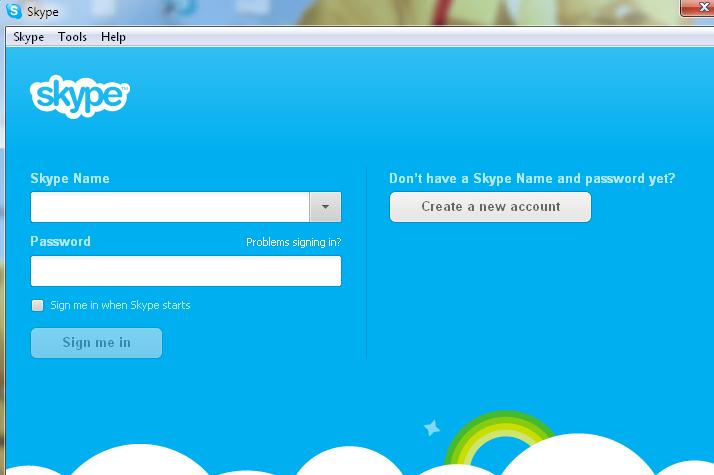This is a detailed screenshot of the Skype login screen. In the upper left-hand corner, the familiar Skype logo and the word "Skype" are prominently displayed against the signature blue background associated with the app. Below this header, there are two text fields: the first for entering a user's Skype name and the second for their password. Once these credentials are provided, the "Sign me in" button, which is initially inactive, will become highlighted, allowing the user to proceed. To the right of the password field, there's an option labeled "Create a new account" for users who need to register a new Skype account. At the bottom of the screen, a checkbox marked "Sign me in when Skype starts" offers users the convenience of automatic sign-in every time the application is launched, by saving their login information.